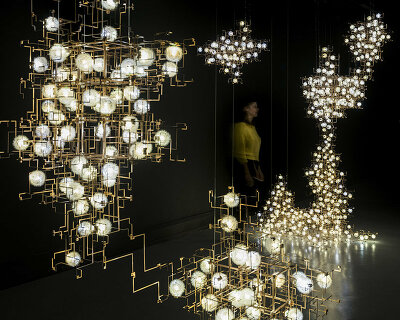In the image, we are inside a darkened room or hall, with discernible hints of walls and possibly a door or a wardrobe. The captivating focal point is an intricate art installation reminiscent of the Infinity mirror exhibit. This installation features a network of golden, angular tubing and framing, interconnected like pipelines, occupying a three-dimensional space. Nestled within these pipes are small, round orbs of light that appear white and yellowish, with a fuzzy glow. These illuminated spheres are arranged in multiple clusters: one prominent cluster on the left side resembling a nest of white eggs, another near the center bottom-right, and additional clumps scattered in the background along the right side and above the middle.

A reflection in a mirror amplifies the visual complexity, showing a side profile of a woman wearing a yellow t-shirt and black pants. She appears slightly blurred, adding a dynamic element to the static brilliance of the light orbs. The overall arrangement of the lights and metal structures creates an arresting visual impression, with some patterns evoking the appearance of chandeliers suspended within the dark space.